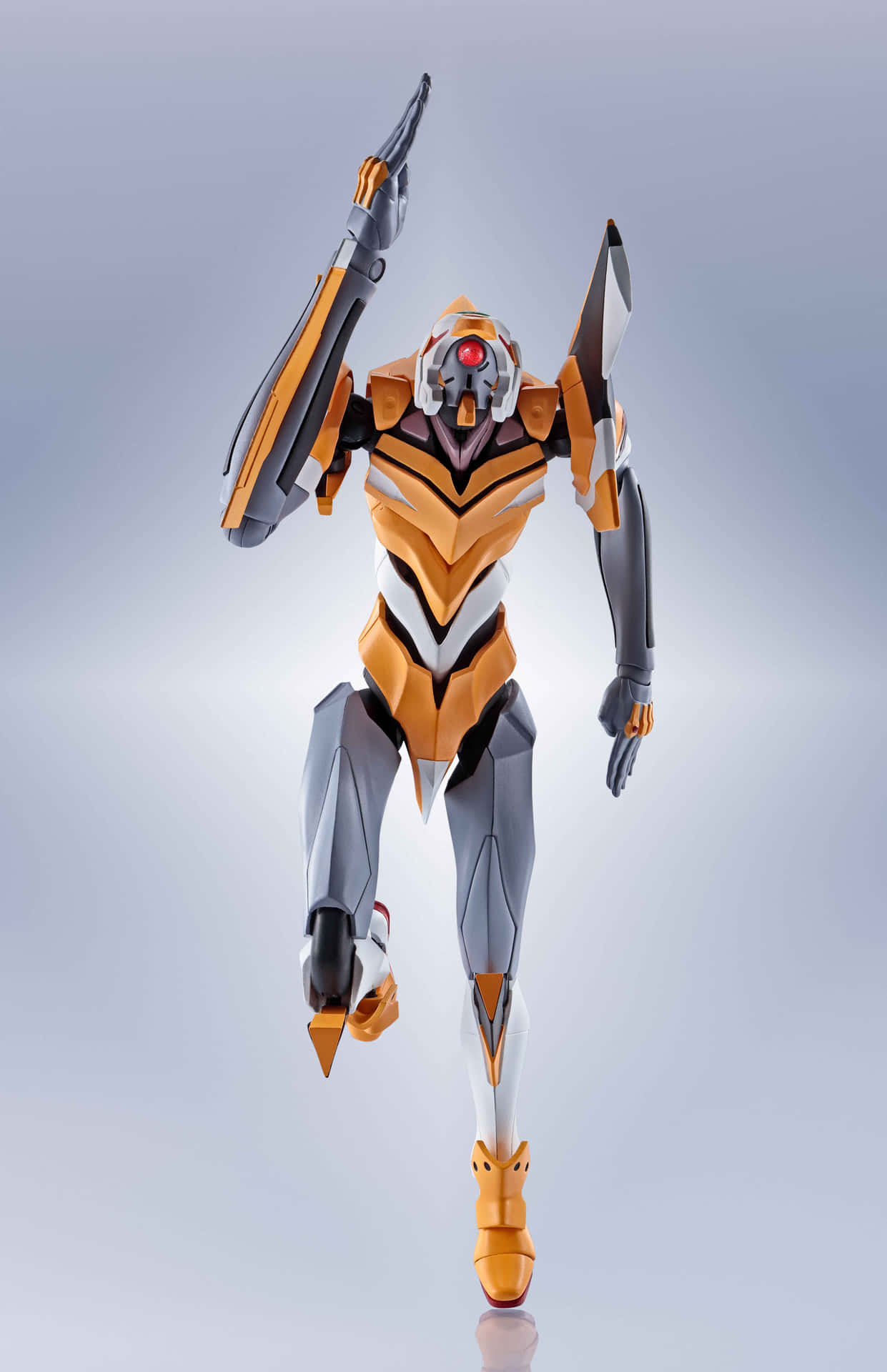In the center of the image, a vividly colored, ultra-thin figurine resembling a power hero or a robot is depicted in a dynamic running pose. This figure is positioned against a backdrop that transitions from dark gray at the top to light gray at the bottom with a distinct white strip cutting across, which resembles a light source behind it. The figure itself is meticulously detailed with a dog-like face featuring a single bright red eye and no other facial features, giving it an intensely robotic appearance.

The torso is adorned in a striking pattern of orange, black, and white V-shaped formations, evoking the imagery of a hornet. The elongated arms, jointed at the elbows, amplify its mechanical design—the left arm elevated above its head, suggesting motion, while the right arm extends backward, elbow up, fingers pointing downwards. Both forearms are predominately gray, accented with orange stripes and black shoulder blades.

Its legs are intricately designed - the left leg bent at the knee and lifted, capturing the essence of movement with the toe pointing downward, while the right leg is firmly planted on the ground. Composed of segmented gray parts, the calves are notably white, adding to its variegated appearance. The shoes, crafted from the same plastic-like material as the body, are orange and segmented, with an elongated section near the ankle.

In summary, this highly dynamic and detailed image showcases a power hero-robot hybrid caught in mid-run, characterized by its vibrant orange, black, white, and gray color scheme, precise joint articulation, and futuristic armor-like construction, all set against a minimalist gradient background.